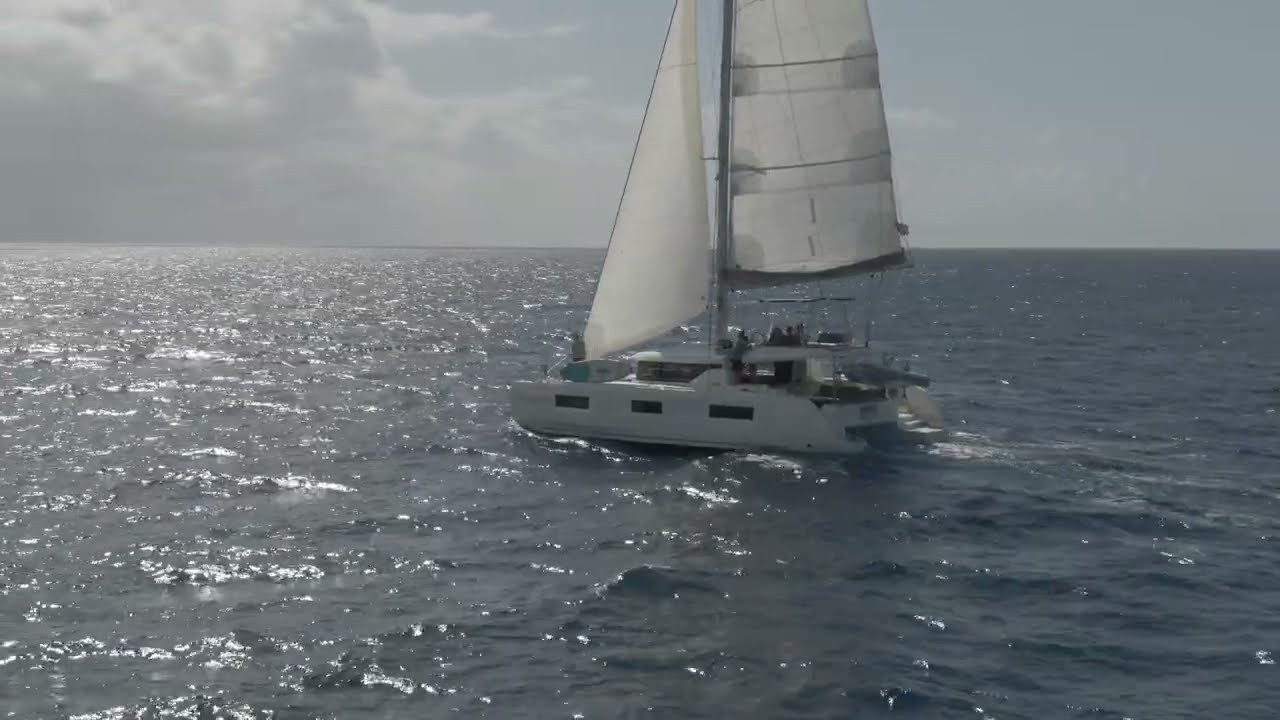The image depicts a large white sailboat, which resembles a cabin cruiser or yacht, positioned centrally in a vast, choppy, grayish-blue body of water. The water is sprinkled with sparkling reflections, especially more pronounced on the left side, possibly due to sunlight, even though the sun itself isn't visible. The boat, characterized by its three windows along its hull and a prominent upper deck area, features two white sails—one at the front and a larger one behind it, both rising from a central mast. The upper part of the boat appears to have a second story or some kind of room, possibly an indoor space or helm area where the captain would be. There are a few indistinct figures on the boat, though the details are blurred due to distance. The sky in the background displays contrasting conditions: dense white clouds and a haze suggesting rain on the left, transitioning to a clearer blue expanse on the right. No land is visible in the scene, emphasizing the expansive and isolated setting of this sailboat amidst the restless waters.